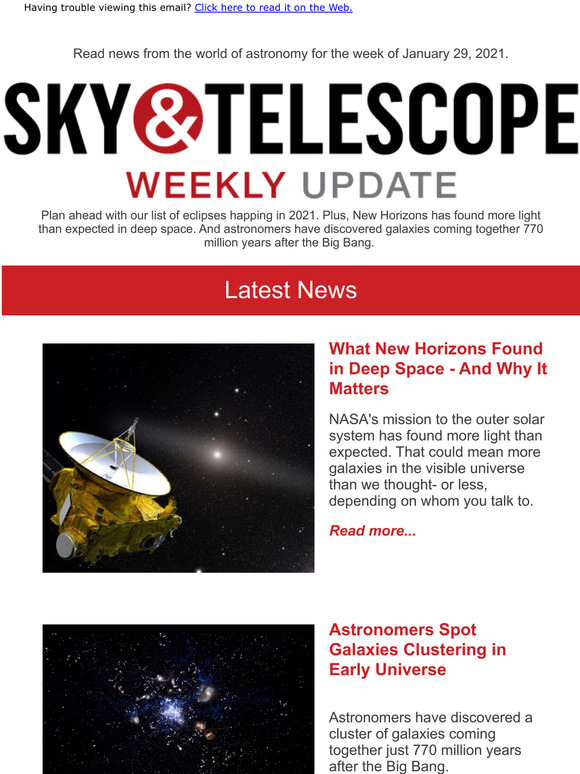The image is a newspaper clipping with a clean white background. At the top, it features a small prompt in plain black text: "Having trouble viewing this email?" To its right, a clickable link in blue text reads, "Click here to read it on the web."

Below this section, the text announces, "Read news from the world of astronomy for the week of January 29, 2021." The main title, "Sky & Telescope," is prominently displayed in large black letters. The ampersand is uniquely styled in white within a red circle.

Beneath the title, the subheading "Weekly Update" uses red for "Weekly" and grey for "Update." Following this, the text entices readers with upcoming astronomical events and discoveries: "Plan ahead with our list of eclipses happening in 2021: New Horizons has found more light than expected in deep space, and astronomers have discovered galaxies coming together 770 million years after the Big Bang."

A noticeable red banner follows, marked with "Latest News" in white text at its center. Underneath this, positioned to the center-left, there is a vivid image of space featuring a large yellow satellite floating against a starry backdrop.

To the right of the satellite image, the headline in red states, "What New Horizons Found in Deep Space—And Why It Matters." Below it, a description reads, "NASA's mission to the outer solar system has found more light than expected. This could mean there are more galaxies in the visible universe than previously thought—or fewer, depending on whom you talk to." A red "Read More" link is situated beneath this text.

The second article features an image of space showcasing a luminous blue nebula surrounded by bright stars against a black void. To the right of this image, the headline in red reads, "Astronomers Spot Galaxies Clustering in Early Universe." Below that, black text elaborates, "Astronomers have discovered a cluster of galaxies coming together just 770 million years after the Big Bang." 

This completes the detailed portrayal of the newspaper clipping image.